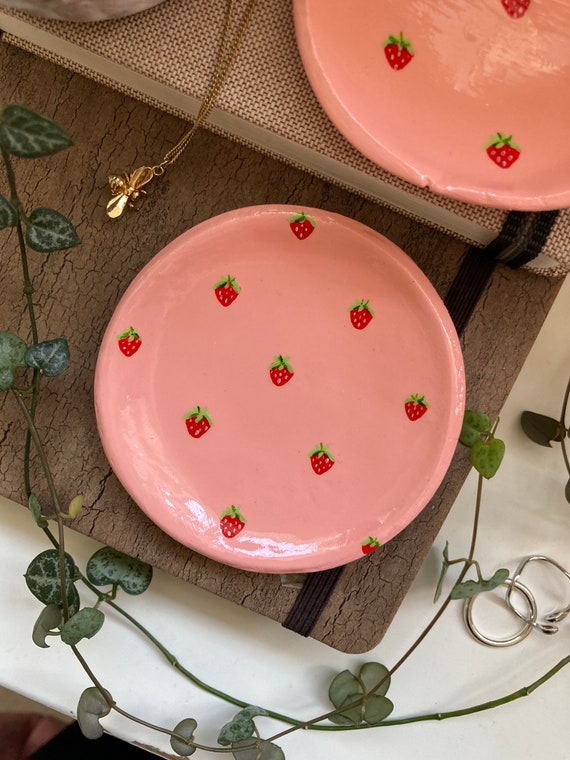The image depicts a detailed and charming summer outdoor tablescape scene. At the center is a rustic brown and white woven surface, resembling a book, supporting two soft pink plates adorned with a repeating pattern of nine imprinted strawberries. The table itself appears to be light-colored, possibly white, with a delicate vine of ivy draped across, adding a touch of natural elegance. Draped gracefully over the upper plate is a golden chain, culminating in a bee-shaped pendant. To the right, two silver rings lie interlocked, contributing an extra layer of intrigue to the composition. The scene is a harmonious blend of textures and elements, creating a visually captivating and serene setting.